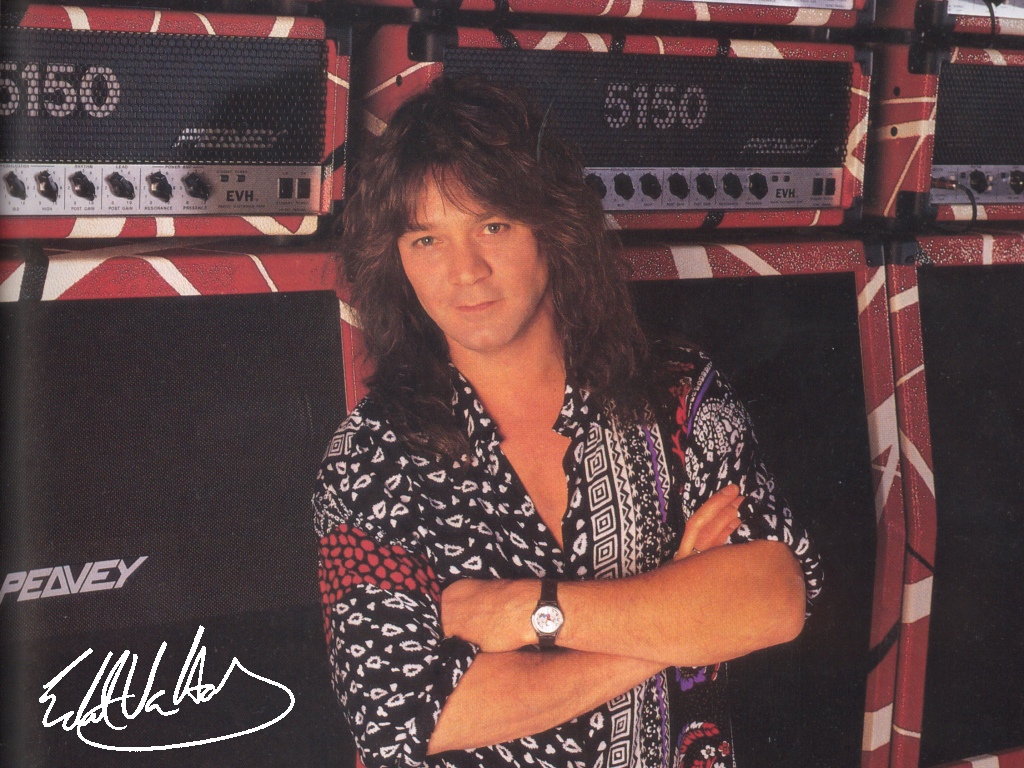The photograph captures what appears to be musician Eddie Van Halen, centered in the frame. He is visible from the waist up, standing confidently with his arms crossed in front of his chest. His long, shoulder-length brown hair is slightly curly with bangs, lending a poofy appearance. Eddie is wearing a partially unbuttoned black shirt adorned with various geometric white designs and red patterns on the sleeves. On his left wrist, he sports a black wristband watch with a white face featuring a cartoon character, and a gold ring is visible on the ring finger of his other hand. Behind him, there are multiple tall stage speakers and amplifiers stacked in three rows, colored in black, red, and white trims. Notably, one of the amps bears the number "5150" at the top, and at the bottom left of the image, Eddie Van Halen's white signature is visible. He gazes directly at the camera with a subtle smirk, and his blue eyes hint at a sense of playful confidence.